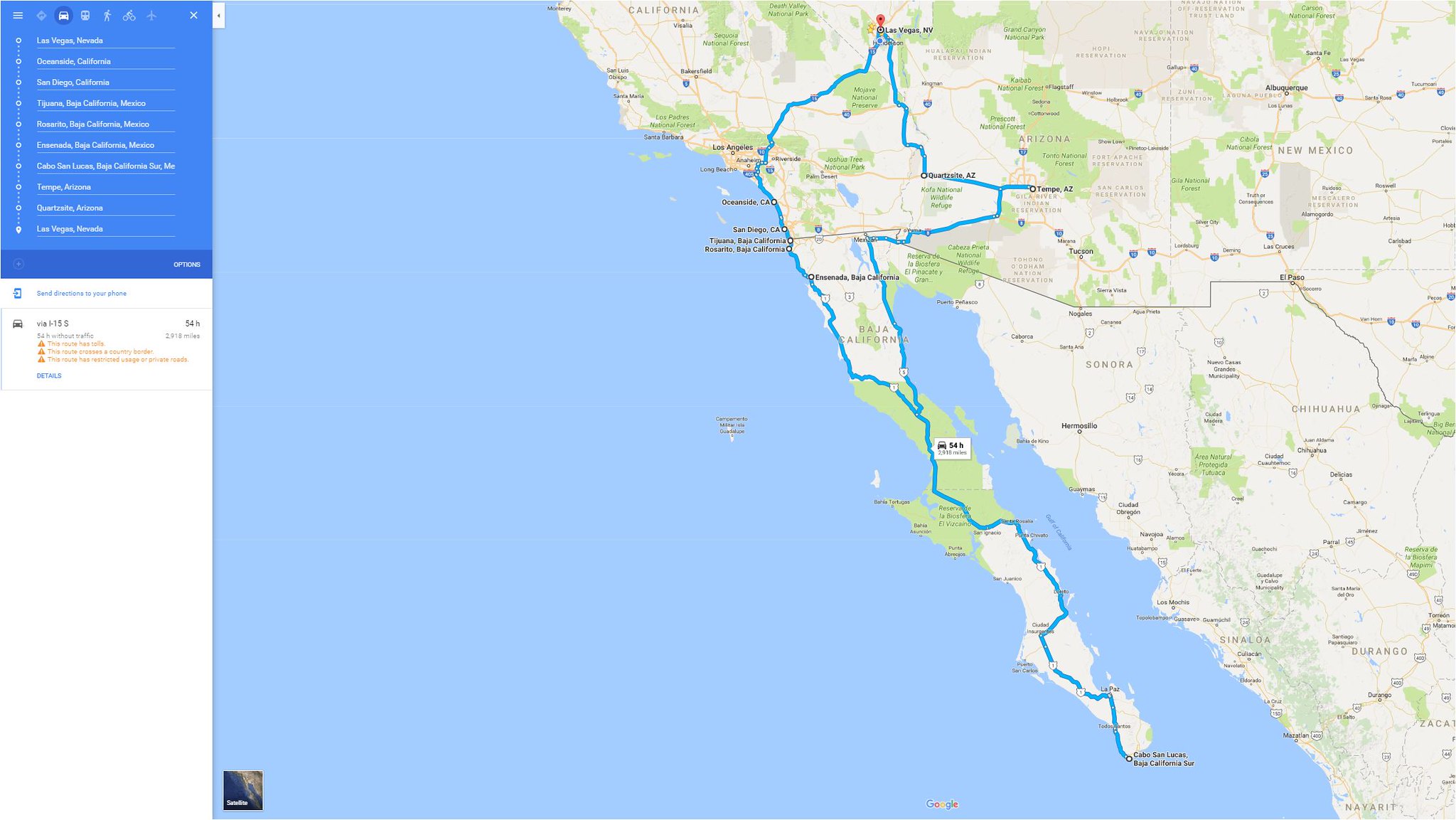The image displays a zoomed-out view of a Google Maps journey, detailing an extensive road trip starting from Las Vegas and stretching all the way down to the southern tip of Baja California. The path continues traveling back up north along the coast of California, passing through San Diego, Los Angeles, Palmdale, and Lancaster, eventually looping back to Las Vegas. The map's background is an off-white color, with the coastline and cities depicted in light brown and green hues. The trip route is marked by a distinct light blue line, providing a clear visual of the planned travel itinerary through various key locations. The left side of the image shows blue representing the coastline, and the detailed route traverses multiple cities and regions, suggesting a comprehensive and scenic drive covering both Mexican and American territories.